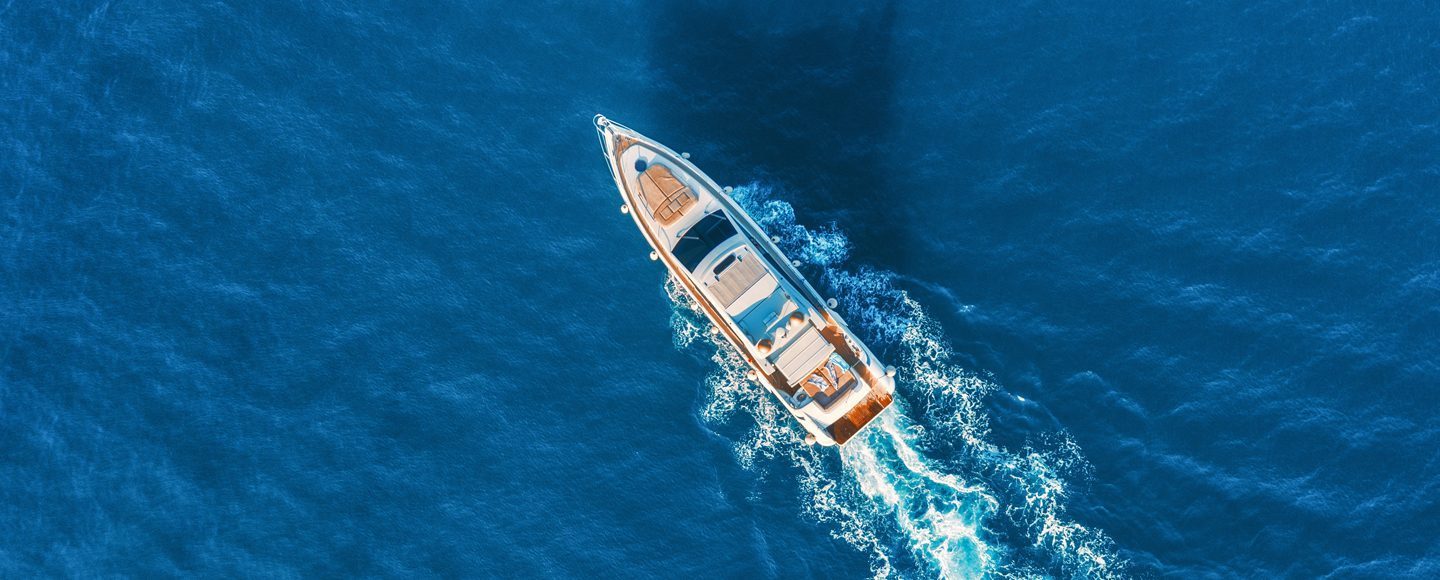This is an aerial view of a small luxury yacht, white with brown trim, elegantly cruising through a bright blue ocean. The ocean water is vibrant, with light wavy lines indicating the movement of waves beneath the yacht. The boat is heading to the upper left, with a white wake trailing behind it, suggesting its motion through the water. The yacht features a top deck with a lounging area and a captain's lounge, indicative of its luxurious nature. A brown and tan canopy casts a shadow over part of the boat, hinting at added comfort for its passengers. The front of the yacht has a tan object and a dark circle, which could be navigational equipment, and the windshield is equipped with two wipers. The back of the boat, constructed from wood, adds a touch of classic elegance with brown and tan hues. Overall, the scene is bathed in sunlight, reflecting off the boat and emphasizing that it is daytime. Notably, there are no people visible aboard the yacht, focusing the viewer's attention on the vessel and its serene oceanic surroundings.